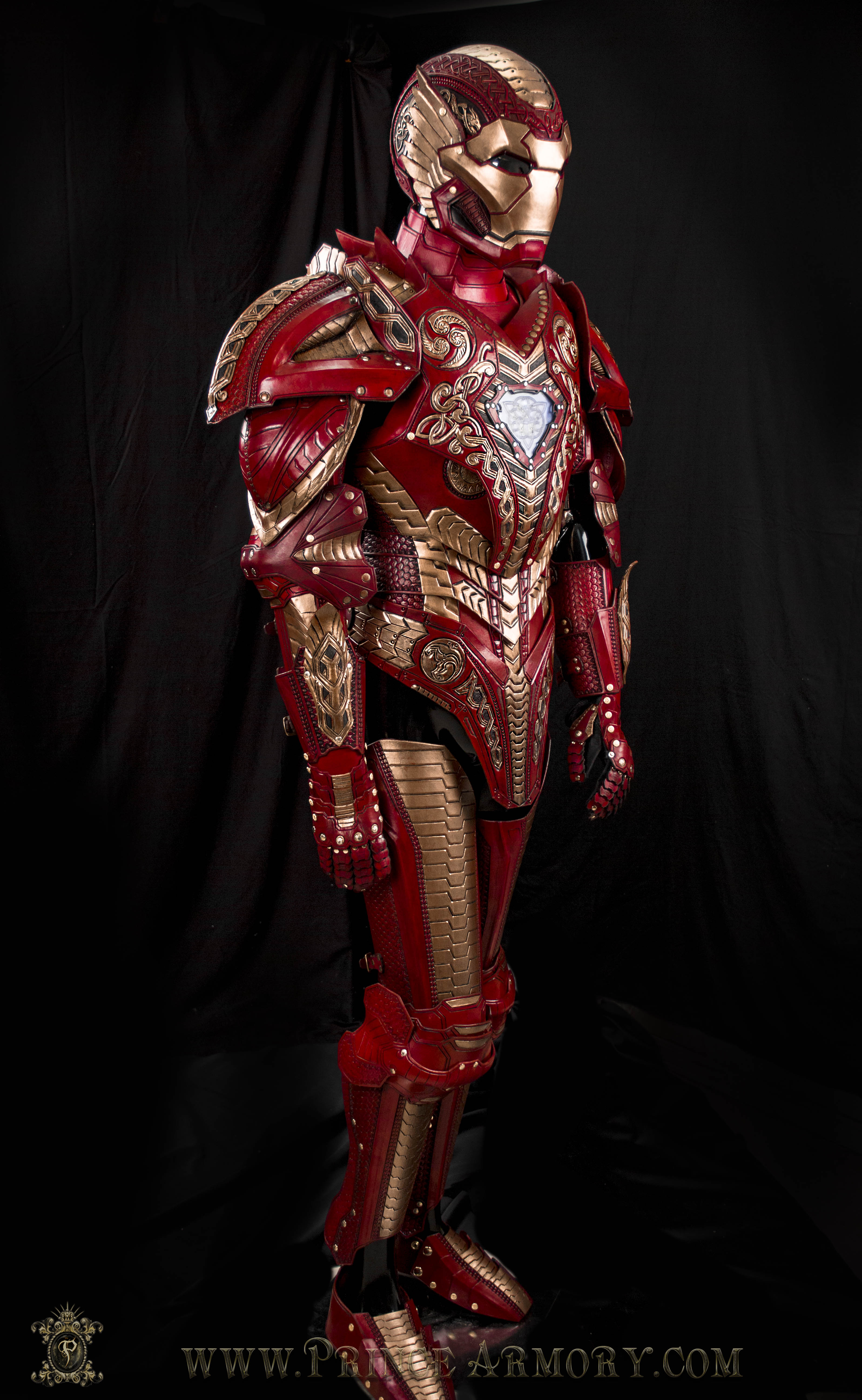The image showcases a custom-made Iron Man suit set against a solid black background. The armor is predominantly red with intricate golden details. The helmet features a brass-colored faceplate with golden stripes, including one running down the center of the forehead. Gold accents extend around the ears and shoulders, creating ornate patterns that suggest a diamond shape in the center of the chest. The arms and legs are fully armored, with golden stripes running down the thighs, shins, and feet, giving the outfit a mechanical and highly detailed appearance. The neck is protected by what appears to be red scales, and the shoulder areas have epaulet-like designs. The entire suit, from the breastplate to the codpiece, is meticulously crafted with additional golden snake-like lines on the stomach. At the bottom of the image, there is a faint inscription that reads "www.princearmory.com." Overall, the suit is a unique and elaborate variation of the original Iron Man armor, complete with detailed gold etchings that set it apart.